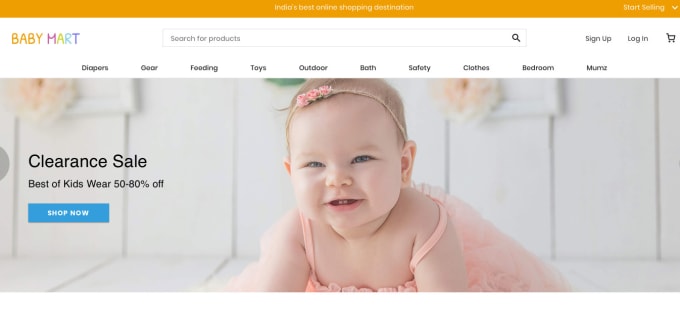The image features a promotional banner for an online shopping platform:

At the top, an orange bar spans the width of the image, with white text in the center reading "India's Best Online Shopping Destination." To the right, there is a "Start Shopping" prompt accompanied by a small down arrow.

Below this, on a white background, the text "Baby" appears in orange on the left side, followed by "Mart" arranged in a colorful sequence of purple, yellow, white, blue, and purple again. These elements are part of the website's branding.

A white search bar, with the placeholder text "Search for Products" in gray, is positioned centrally. To its right are links for "Sign Up," "Log In," and a shopping cart icon.

A black navigation bar lists various categories: Diapers, Gear, Feeding, Toys, Outdoor, Bath, Safety, Clothes, Bedroom, and Mums (stylized as "M-U-M-Z").

The main content showcases a stock photo of a white baby with blonde hair, seated in a white crib, smiling with two small teeth visible. On the left side of the photo, black text reads "Clearance Sale," "Best of Kids Wear," and "50-80% off." Below this, a blue "Shop Now" button with white text invites further browsing.

The banner's detailed layout aims to guide users through different shopping options and promotions.